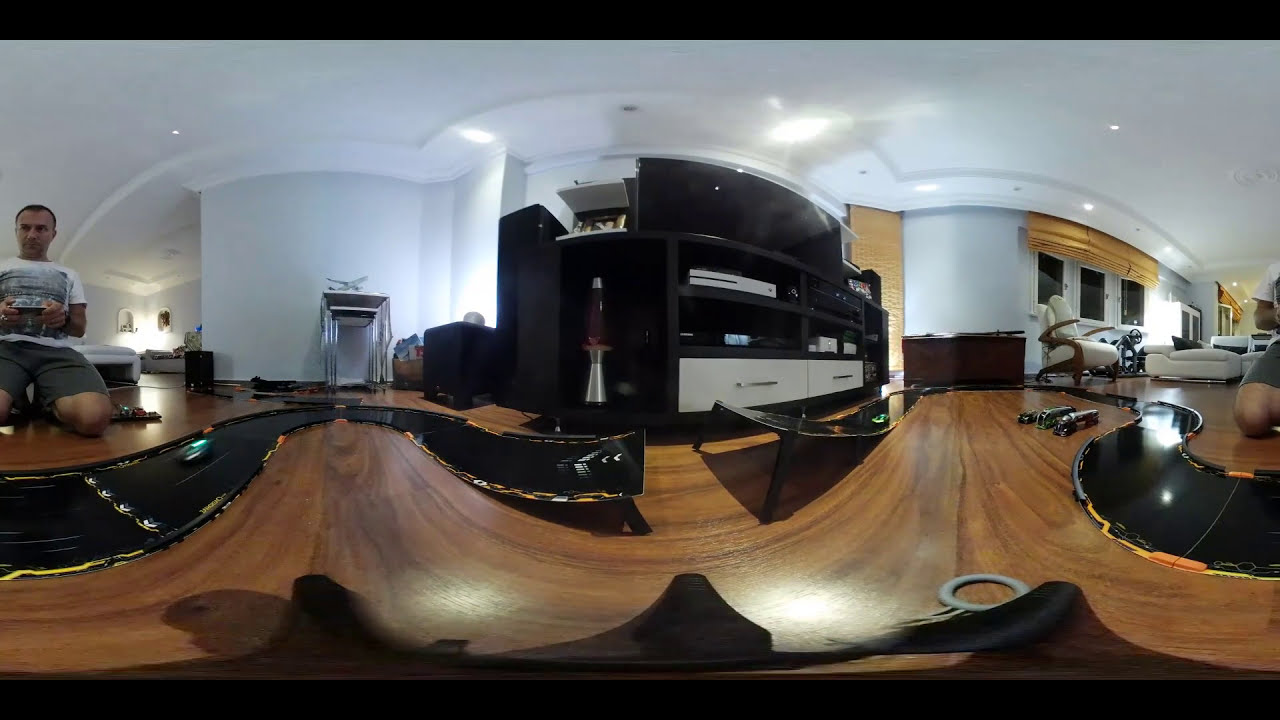The image showcases a panoramic view of a modern living room, creating a wavy effect as the middle portion is closer to the viewer. The room features a white ceiling with built-in lights and beautiful hardwood flooring. Dominating the center of the floor is a large, black and curvy racetrack that stretches across the space. A man, dressed in a t-shirt and dark-colored shorts, is kneeling on the wooden floor, engrossed in playing a video game with a controller in his hand. To the left of the racetrack, there's a black entertainment center topped with a large TV and a distinctive large lava lamp, and equipped with two sizeable white drawers at the bottom. The background of the room includes modern white furniture—a couch and a chair—and a brown dresser, with windows that allow natural light to enter the space. The overall design of the room is circular and contemporary, characterized by a harmonious blend of black, brown, and white tones.